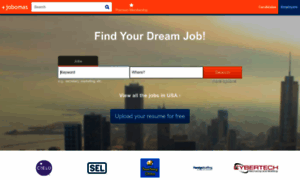A screenshot of the Jobomas website highlights its logo, which resembles a plus sign, prominently displayed. At the top of the page, "Find Your Dream Job" is written in large white letters, serving as an inviting headline. The site features a user-friendly search area where users can enter keywords and specify the location for their job search, thus allowing detailed filtering based on job descriptions and geographic preferences. Once the search parameters are set, users can click an orange "Search" button to proceed. Additionally, there is a white button labeled "View All Jobs in the USA," offering quick access to a comprehensive list of job postings across the country. Towards the bottom of the page, a blue button encourages users to "Upload Your Resume for Free," simplifying the application process. The screenshot also shows logos from various companies like Cybertech, Uber, and SEL, suggesting partnerships or affiliations with Jobomas to offer more job opportunities.